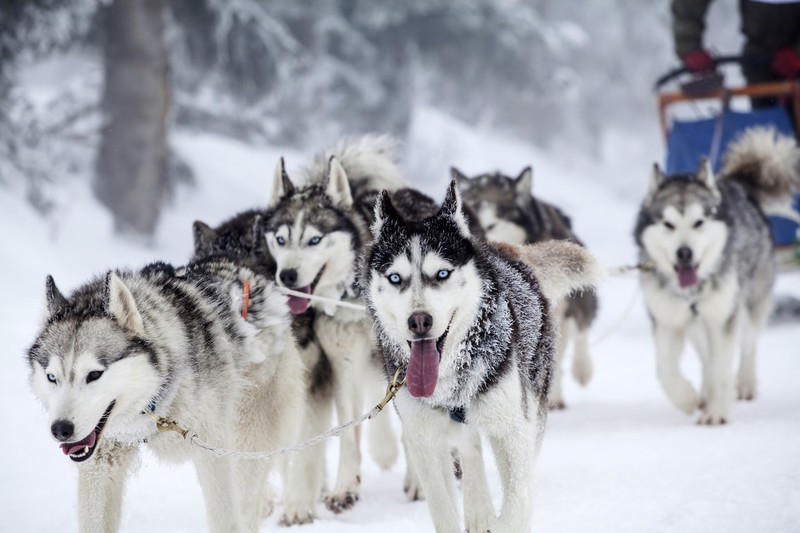The photograph captures a lively and picturesque scene set in a snowy, mountainous region resembling places like Alaska or Colorado. The central focus is on a pack of six husky dogs, all chained together and energetically pulling a sled. These huskies, characterized by their black and white coats, bushy tails, and striking blue eyes, mostly have their tongues out, appearing joyful and well-suited for the cold environment. One husky on the bottom left notably has one blue eye and one darker eye. The dogs, some of whom are dusted with snow, stand out vividly against the white, snowy ground.

In the blurry background, trees and mounds of snow are visible, enhancing the wintery ambiance. The sled, with its blue tarp and orange frame, is being guided by a person, only partially visible, clad in a jacket and distinctive red gloves. This person is positioned towards the right-hand side of the image. Despite the blurred backdrop of snow-laden trees, the scene is imbued with a sense of motion and adventure, showcasing the dogs’ spirit and the serene, frosty landscape around them.